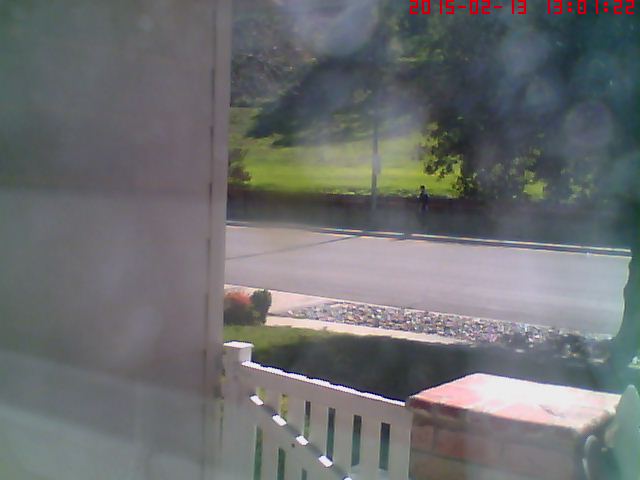The image captures the outdoor view seen from a Ring Cam, likely mounted inside a house and overlooking the street. The foreground features a white picket fence and a brick pedestal, with a patch of green grass by the sidewalk. The sidewalk itself is bordered by gravel and a cobblestone pathway. On the left side, a wall from the house is visible, and the street beyond is void of automobiles. Across the street, more green grass can be seen alongside tall trees on the right-hand side. The image quality suggests it was taken with an older digital camera, and it is time-stamped with "2015-02-13 13:01:22" in red digits at the top. In the distance, a man is walking along the sidewalk, captured by the motion sensor. There is also a sign visible on the sidewalk.